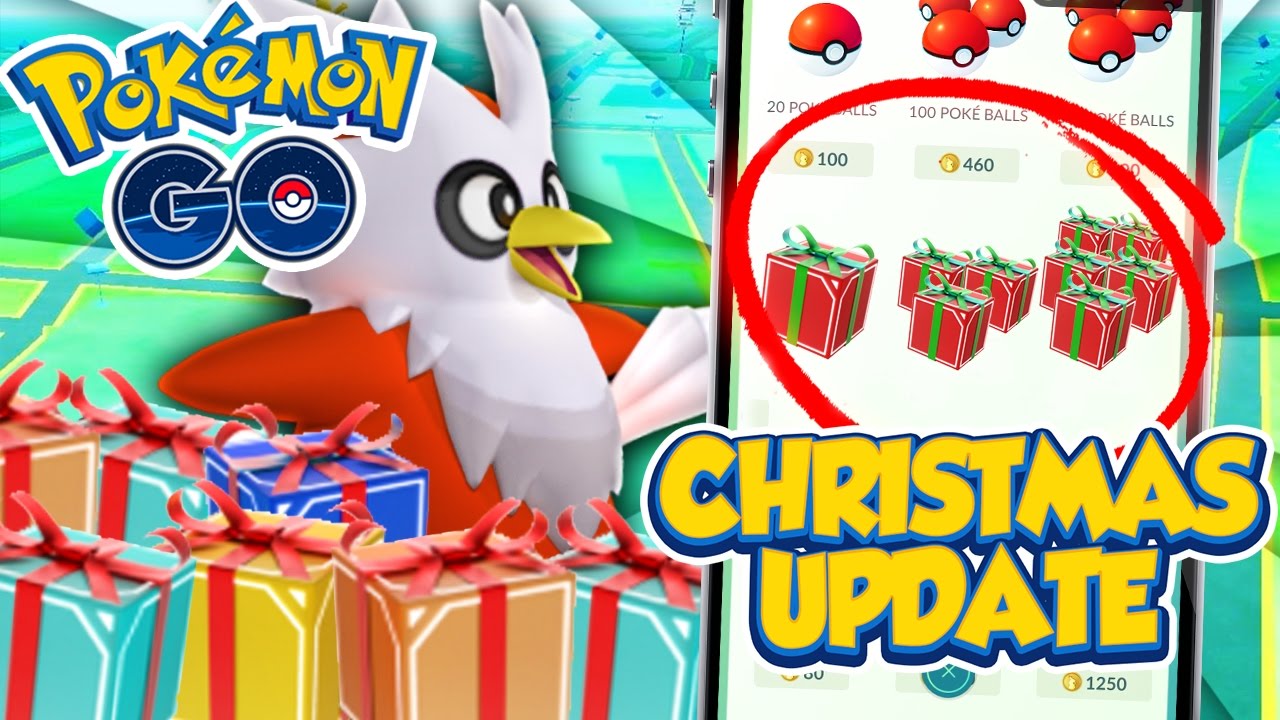This advertisement showcases a festive Christmas update for Pokémon Go. On the right-hand side, a tablet screen is prominently displayed. At the top of this screen, there is a single Pokémon ball, followed by two rows of three Pokéballs each, adding up to a total of seven Pokéballs. Below the tablet screen, there are several packages of Christmas presents, beautifully wrapped in red paper with white designs and adorned with elegant green bows. These presents are grouped in sets of one, three, and five, and they are encircled with a bold red outline. 

A striking yellow text stretches across the screen and even extends out of the tablet, announcing the "Christmas Update." On the left-hand side of the advertisement, the iconic "Pokémon" logo can be seen at the top, followed by "Go" and the distinctive Pokémon bird symbol. Beneath this, there are more Christmas presents wrapped in an array of colors including tan (peach), light blue, dark blue, yellow, and additional light blue. The entire background is a soothing aqua color, adding to the festive and vibrant atmosphere of the advertisement.